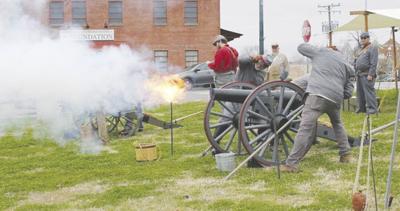In this modern photograph capturing a Civil War reenactment, four men dressed in period-appropriate gray uniforms are operating vintage cannons. The scene is set in a small grassy field, part of the downtown area of a small town. The grass shows signs of wear, with brown patches scattered throughout. In the foreground on the right, a cannon is captured mid-fire, producing a dramatic burst of orange flame and a cloud of thick smoke. This firing cannon is gray and positioned to the left.

Two men are positioned on either side of the firing cannon, both plugging their ears against the deafening blast. In the background, two more participants in gray uniforms look on. One additional figure stands out, wearing a bright red shirt with suspenders and gray pants, adding a vivid contrast to the scene. Besides the red-shirted man, there is another indistinct figure further in the background, also equipped with period-style attire and a hat.

Behind this reenactment, modern elements blend into the historical tableau. A red stop sign is clearly visible, along with a parked car. Across the street, a two-story red brick industrial building looms, featuring partially obscured signage above its doorway. This juxtaposition of historical re-creation against a contemporary backdrop highlights the anachronistic charm of the event.